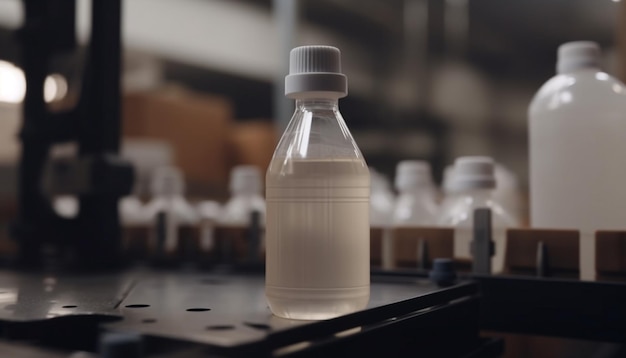This horizontal image appears to be taken inside a factory or lab and features a prominent close-up of a plastic bottle sitting on a black metal shelf with holes in it. The bottle, which is smaller than a 16-ounce bottle and more likely around 8 to 12 ounces, is almost completely filled with an opaque, milky white liquid. It has a gray screw-on cap that contrasts with other white caps visible in the scene. 

In the blurred background, there are several other bottles of various shapes and sizes, including empty ones and some partially visible larger bottles to the right edge of the picture. These bottles also feature caps, mostly white but differing in style. The setting suggests a storage area within a bottling factory, covered in subdued lighting that casts a dark overall tone across the image.